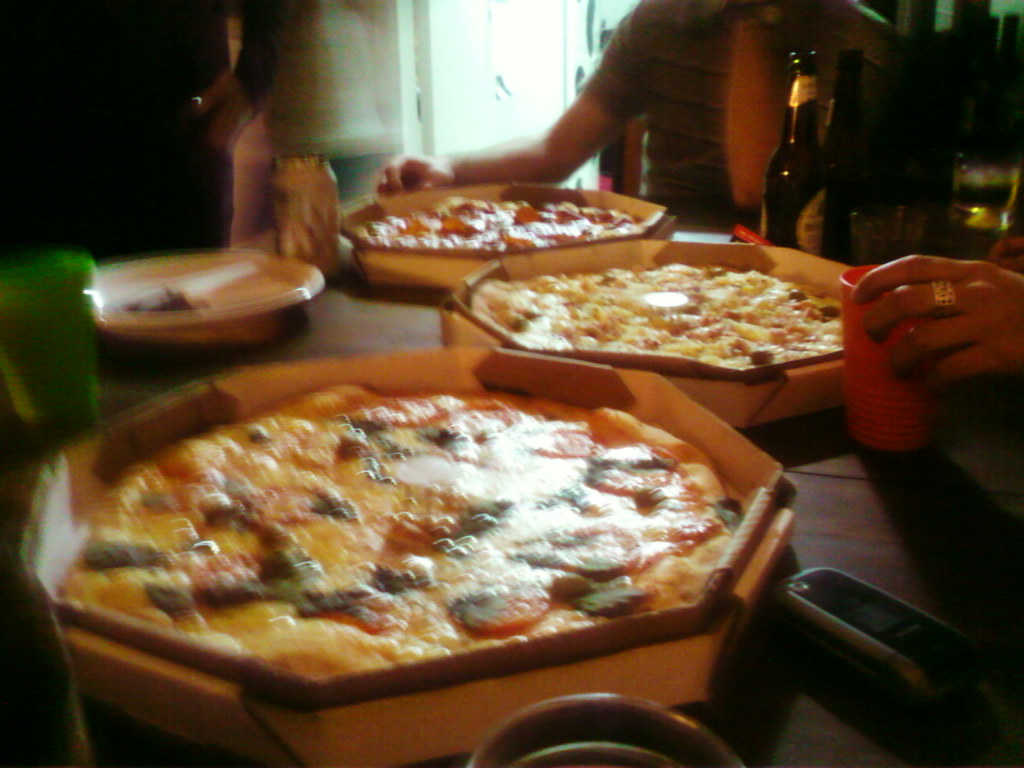This image depicts a slightly chaotic, yet inviting gathering around a rustic, round wooden table with mismatched planks. Three distinct pizza pies are placed on elevated cardboard bases resembling a miniature stadium tower setup, adding height and depth to the presentation. Despite the blurriness of the photo, it’s evident that one pizza in the foreground is topped with pepperoni and possibly sausage and green peppers. Another pie appears to feature greens, tomatoes, and perhaps pineapple, while the third pizza, farther back, seems loaded with pepperoni. Surrounding the main attraction are several beverages: a prominent bottle of beer towards the back, a green cup on the left, a red plastic cup held by a hand adorned with a gold ring, and a partially visible flip phone next to a section of a glass. An arched window or glass door in the background casts a bright, glowing light into the scene. The people gathered wear casual attire, including one person in a cream and brown shirt, adding to the relaxed, home-like atmosphere. Plates and faint food piles suggest a feast well underway.